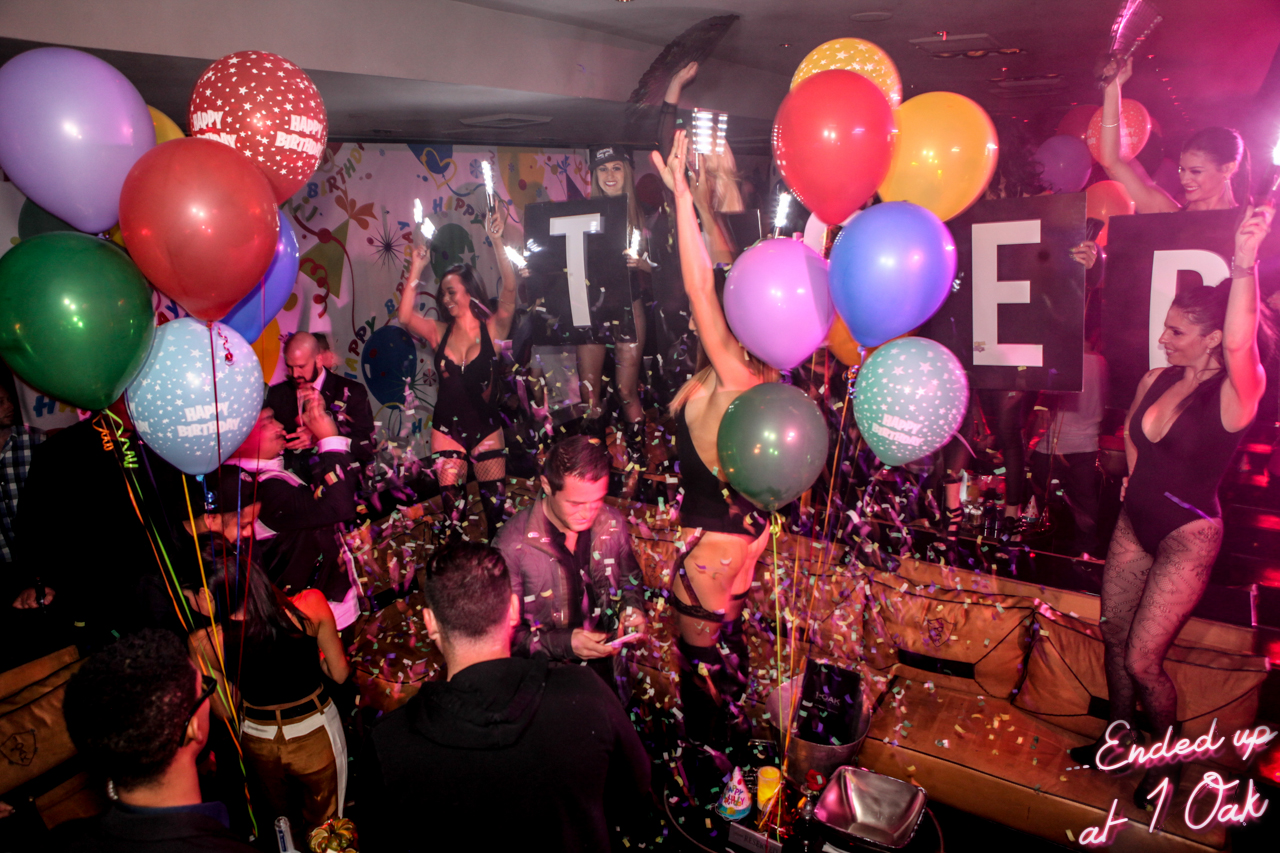This lively photo captures the exuberant scene of a birthday celebration at what appears to be a nightclub named "One Oak," as indicated by the neon sign in the bottom right corner. In the center of the image, a man is focusing on something in his hands, possibly a gift or his phone, surrounded by a boisterous crowd. Multi-colored balloons—purple, red, green, yellow, and blue—embellished with streamers are tied to various locations in the room, alongside balloons reading "Happy Birthday."

Confetti fills the air, adding to the festive atmosphere. Several women, likely performers, dressed in unitards and black stockings, are energetically dancing with their hands raised, standing atop furniture such as tables and a couch. One woman holds a piece of a sign displaying partially hidden letters, seemingly spelling out the birthday person's name, with visible letters "T something something E D." The crowd also includes gentlemen in rather formal attire, one notably balding, and another wearing sunglasses, contributing to an ambiance that merges both casual and possibly business-related interactions. Despite the slightly dated clothing hinting at an 80s or 90s vibe, the party exudes a timeless sense of revelry.